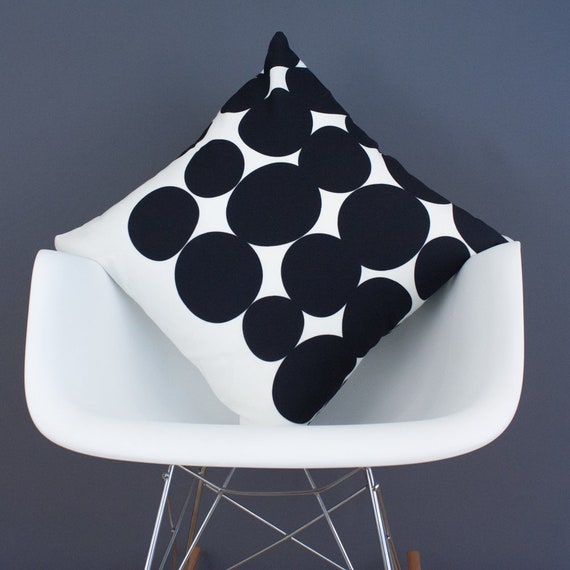The image depicts a modern, white bucket-style chair positioned against a dark grayish-blue wall, creating a stark yet sophisticated contrast perfect for a design magazine or interior blog. The chair features a sleek, molded plastic shell with high, rounded arms and a seat that wraps around the sitter, reminiscent of a director's chair in shape but more sculptural, resembling half of a cup. The chair is supported by a shiny, intricate metal frame combining thin beams and cross-legged components for a contemporary look. A prominent element in the composition is a large, white throw pillow adorned with a pattern of dark navy polka dots arranged in orderly rows. The pillow is placed diagonally, with its corners respectively touching both arms of the chair and one corner pointing downward, almost filling the entirety of the seat. The minimalistic setting, which includes subtle hints of wooden elements barely visible at the image's bottom, emphasizes the artistic and functional blend of modern furniture design.